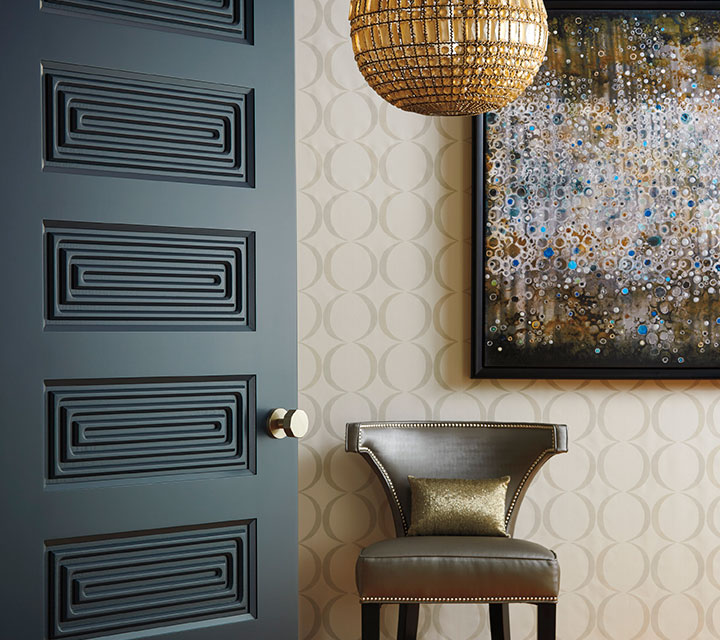This photograph captures a detailed view of a sophisticated interior room. To the left, an ornate, black wooden door—sometimes appearing dark bluish-green under certain lighting—boasts intricate design details with four vertically aligned panels of concentric rectangles, creating a textured 3D effect. The door features a brushed brass knob, which glimmers like gold. Adjacent to the door stands a modern leather chair, studded with brass rivets along its borders, and adorned with an oblong, glittering gold pillow. Above the chair, a chandelier hangs, resembling yellow or brass-colored crystal with orange accents, casting a warm glow in front of a beige wallpaper. The wallpaper itself is patterned with repeating vertical lines of darker taupe circles. Enhancing the aesthetic appeal, an abstract artwork in a dark brown to black frame is positioned above the chair. The painting has a brown background splattered with glittering accents of cyan, blue, orange, white, gray, and black, adding a vibrant touch to the refined setting.